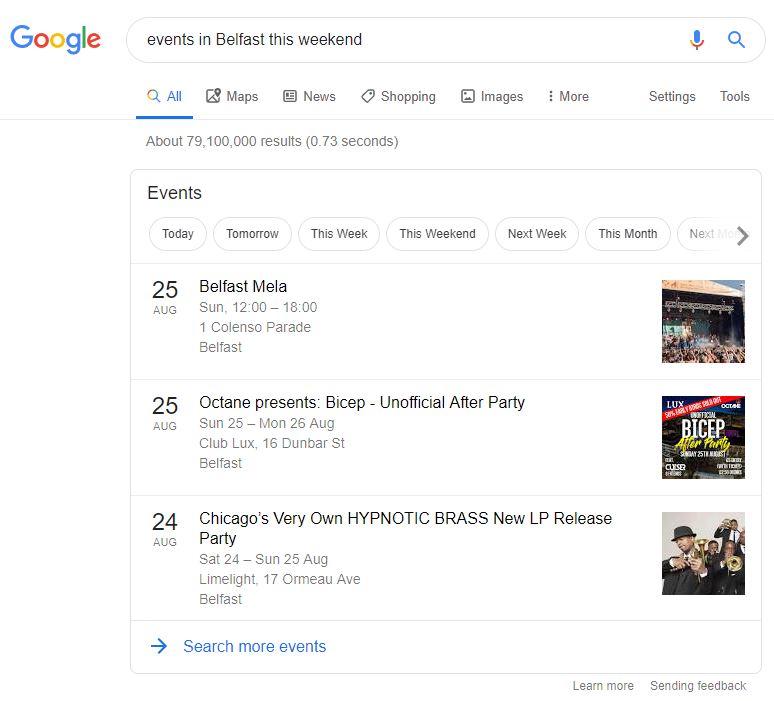Screenshot of Google Search Results Page

The image captures a Google search results page with a clean, white background. In the top left corner, the colorful Google logo stands out. Beside it, the search field, outlined in a black oval, contains the text "events in Belfast this weekend." At the right end of the search field, there are microphone and magnifying glass icons. 

Below the search bar, a row of options is displayed: 

- "All" accompanied by a magnifying glass icon
- "Maps" with a map icon
- "News" with a newspaper icon
- "Shopping" with a shopping tag icon
- "Images" with a photo icon
- "More" represented by three vertical dots

To the far right of this row are the "Settings" and "Tools" options. Directly beneath, in gray font, it indicates the search results: "About 79,100,000 results in 0.73 seconds." 

Following this, the page introduces section titles in black font, starting with "Events." Below this title, clickable filter bubbles offer selections such as "Today," "Tomorrow," "This Week," "This Weekend," "Next Week," "This Month," and "Next Month."

The first entry listed is for the Belfast Mela, scheduled on the 25th of August, running from 12:00 to 18:00 at 1 Colenso Parade, Belfast.